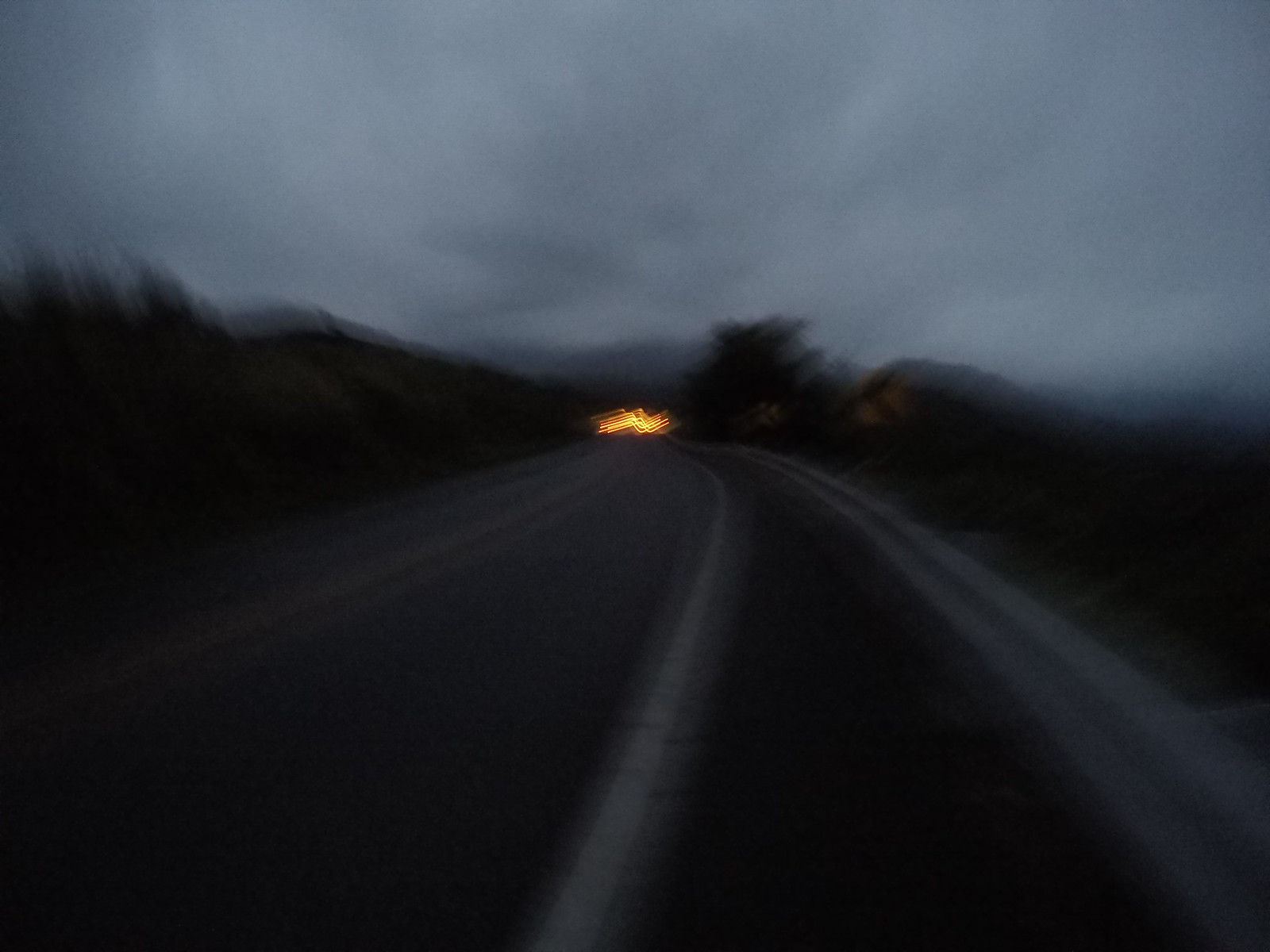The photograph captures a nighttime scene of a two-lane road, slightly blurred in the background, framed within a rectangular landscape format that is only marginally wider than it is tall. Beginning at the bottom edge of the image, the road spans across the lower 10 to 20 percent and then gradually narrows as it recedes towards the vanishing point just above the center. A subtle curve to the left is noticeable, and a prominent white stripe runs along the middle of the road, accompanied by additional stripes on either side.

Dominating the center where the road converges is a peculiar, bright orange zigzag light, resembling a sideways, backward 'Z.' Its exact nature is unclear, but it stands out sharply against the otherwise dark environment, leading one to speculate that it might be a digital artifact added post-processing.

The surroundings are enshrouded in darkness, with vague outlines of dense trees and shrubbery marking the edges of the road. Above, the sky occupies the top third of the image, presenting a medium gray hue suggestive of an overcast night. The horizon is faint and distant, obscured by the nighttime gloom, with the image's primary focus drawn to the enigmatic glowing zigzag.